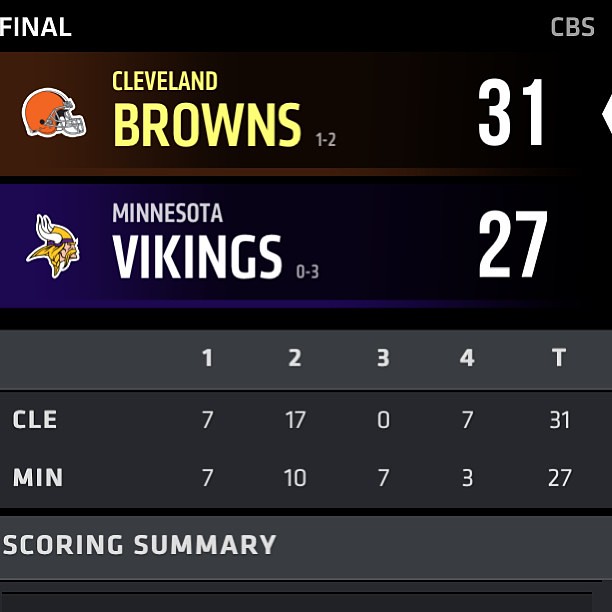This image depicts a detailed scoreboard of a football game between the Cleveland Browns and the Minnesota Vikings, with the final score showing a Cleveland victory at 31 to 27. The word "Final" is displayed prominently in the top left corner, while "CBS" appears in the top right corner. The scoreboard has a black background, except for a gray section at the bottom labeled "Scoring Summary" in white.

The top half of the scoreboard features the team names and details. On the left, with a bright red background, the Cleveland Browns are listed with their helmet logo. Their team name is in yellow text, and their game record is 1 win and 2 losses. They scored 31 points in this game. The right side features the Minnesota Vikings, placed on a blue (or purple) background with their helmet logo in white. Their record shows 0 wins and 3 losses, and they scored 27 points.

The lower part of the scoreboard breaks down the points scored in each quarter by both teams. Cleveland scored 7 points in the first quarter, 17 in the second, 0 in the third, and 7 in the fourth, totaling 31 points. Minnesota scored 7 points in the first quarter, 10 in the second, 7 in the third, and 3 in the fourth, culminating in 27 points. Below this breakdown is the "Scoring Summary" section, highlighting key moments and scores.